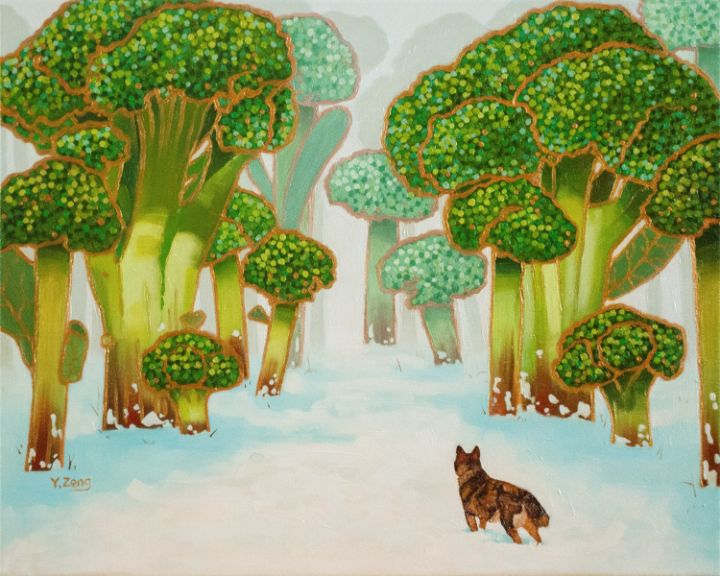This whimsical hand-painted piece showcases a serene, snowy forest where the trees amusingly resemble broccoli stalks. Each tree features a brown base that transitions to yellow and finally to shades of green at the top, adorned with light green and yellow circles. The forest is bordered with brown edges, enhancing its detailed, primitive style. In the foreground stands a highly-detailed, large furry dog, possibly a husky, with its back to the viewer. The dog's alert ears and posture, along with its slightly downturned tail, suggest it is intently gazing into the broccoli forest. The peaceful scene is set against a light blue and white background, evoking a snowy, tranquil atmosphere.